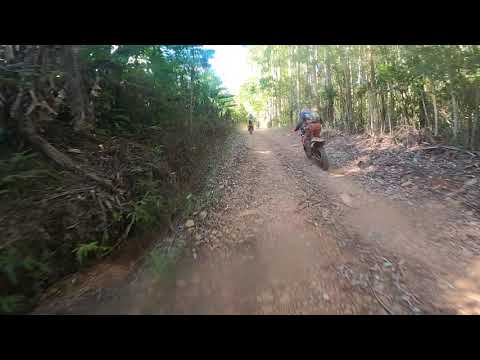The image captures a vibrant outdoor scene set in the middle of the day, showcasing a dirt trail cutting through a forested area. The trail, composed of hard-packed dirt interspersed with rocks and leaves, leads upwards between rows of thin, tall trees. Two motorcyclists, likely dirt bikers, are riding up the trail, moving away from the camera, which seems to be held by a third rider. One of the bikers appears to have a backpack, and a dust trail follows the front rider, indicating they are moving at a high speed. The trees on both sides of the trail grow close to the edge, creating a well-shaded path with sunlight filtering through the canopy ahead. The road shows signs of wear, forming two ruts with debris in the middle. Despite the image being slightly blurry, adding a dynamic feel to the scene, it captures the essence of an adventurous ride through a scenic, forested dirt trail.